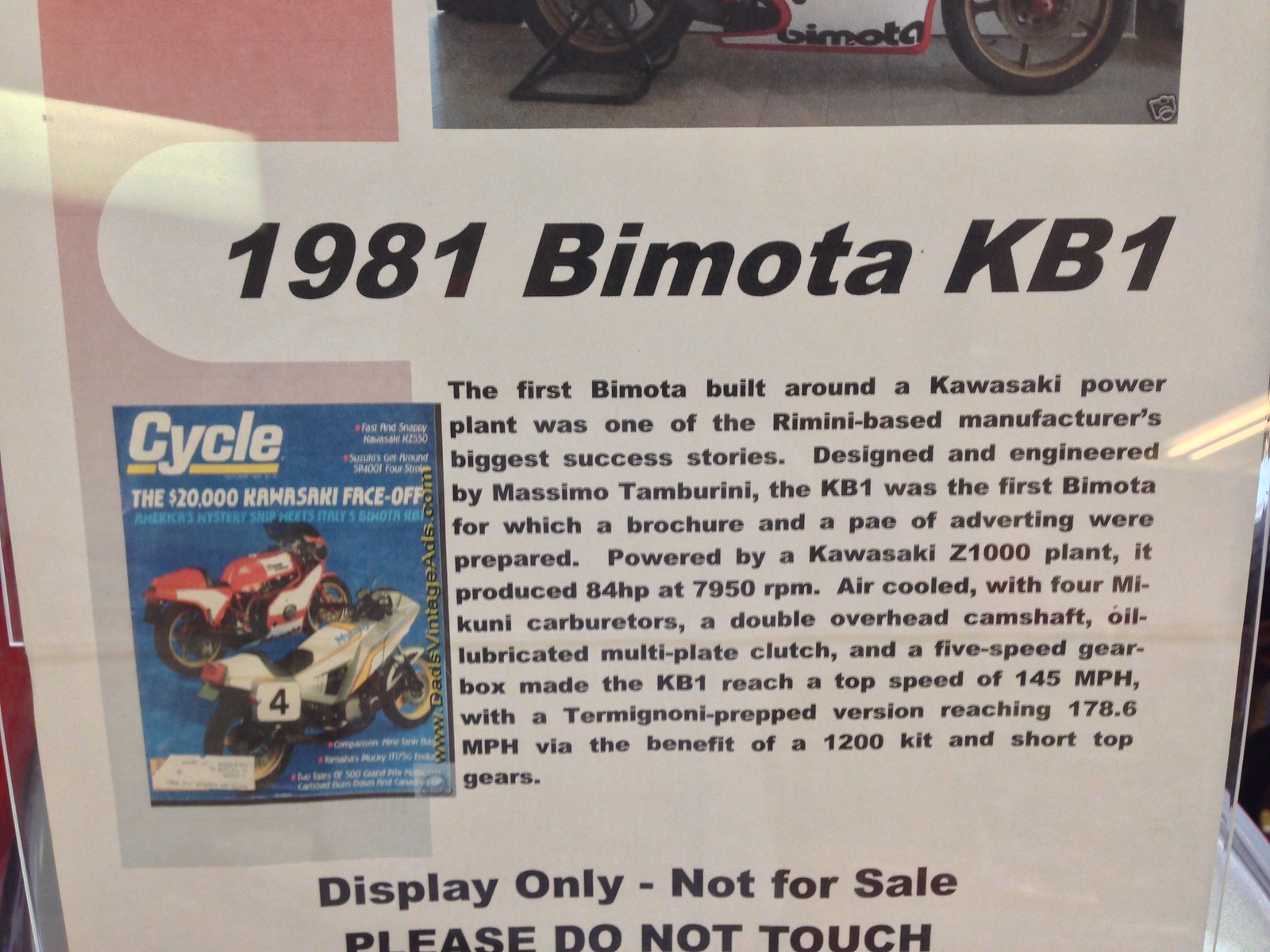This image captures a perfectly square photograph of a display sign featuring the 1981 Bimota KB1, the first Bimota motorcycle built around a Kawasaki power plant. The display, set against a white background, includes various elements emphasizing the motorcycle's significance. At the very top right, partially cut off, are two prominent tires. In the upper left corner, a vertically oriented pink banner transitions into blue, beneath which lies an issue cover of Cycle Magazine, titled "The $20,000 Kawasaki Face-off." The cover showcases two motorcycles: one red and white, and the other white and yellow. 

Directly below, black text highlights the "1981 Bimota KB1," noting it as a major success for the Rimini-based manufacturer. Detailed specifications are provided: designed and engineered by Massimo Tamburini, the KB1 was the first Bimota to feature a dedicated brochure and advertising. It was powered by a Kawasaki Z1000 engine, producing 84 HP at 7950 RPM, and featured air cooling, four Mikuni carburetors, a double overhead camshaft, an oil-lubricated multi-plate clutch, and a five-speed gearbox. The standard model reached a top speed of 145 mph, with a Teramagoni prepped version achieving 178.6 mph thanks to a 1200 kit and short top gears.

Concluding the display, a notice at the very bottom in black lettering reads: "Display Only - Not For Sale - Please Do Not Touch." This detailed advertisement encapsulates the impressive engineering and historical significance of the 1981 Bimota KB1.